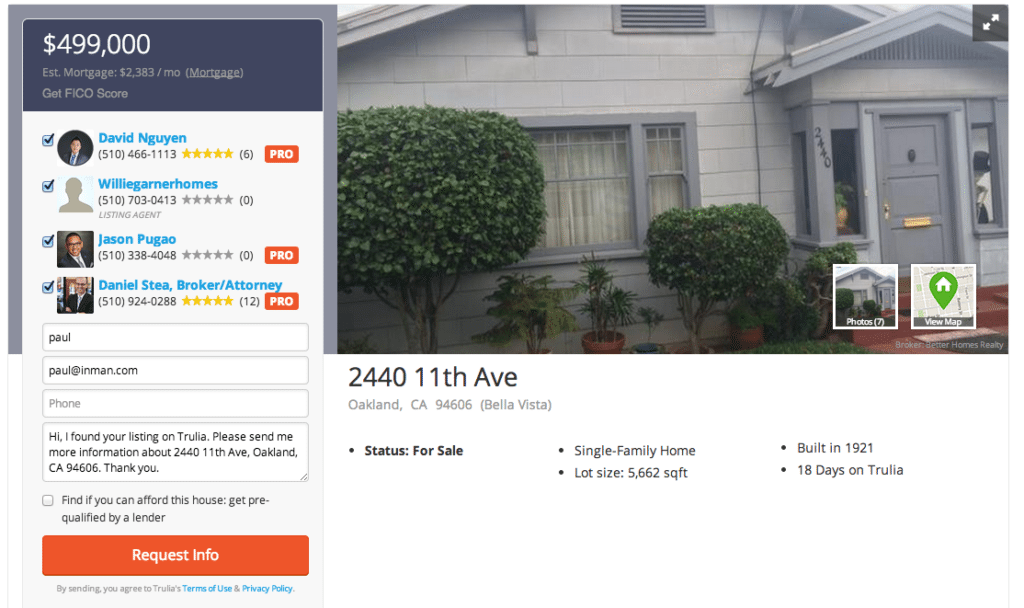This image is a screenshot from a real estate website, specifically Trulia. It captures a small portion of the webpage, primarily focusing on the top-right section. Dominating the top two-thirds of this section is a close-up photograph of the front of a gray-painted house. The window panes and door are painted in a slightly darker gray, complemented by beautifully manicured green bushes positioned on the left and near the front entryway.

Beneath the photo, set against a white background, the address "2440 11th Avenue, Oakland, CA 94606" is displayed, with "The Bella Vista" in parentheses. The status of the property is listed as "For Sale." Two columns of bullet points provide additional details: in the first column, it states "Single Family Home," followed by "Lot Size: 5,662 square feet." In the second column, it mentions the house was "Built in 1921" and notes it has been "18 days on Trulia."

On the left, there's a sidebar with a grayish-blue background at the top, displaying the asking price in large white digits: "$499,000." Below this, written in gray font, is the estimated monthly mortgage, "$2,383 per month," with "Mortgage" underlined, indicating a hyperlink. Further down, it says "Get FICO Score."

The sidebar continues against a white background, listing four real estate agents with their star ratings. The top agent, David Nygen, has a five-star rating, as does the bottom agent, Daniel Stea (pronounced S-T-E-A), who is identified as a broker/attorney. A request information form is also visible, featuring fields for the name, email address, and phone number. The pre-filled message states, "Hi, I found your listing on Trulia. Please send me more information about 2440 11th Avenue, Oakland, CA, 94606. Thank you." Below the form is an orange button labeled "Request Info" in white font.